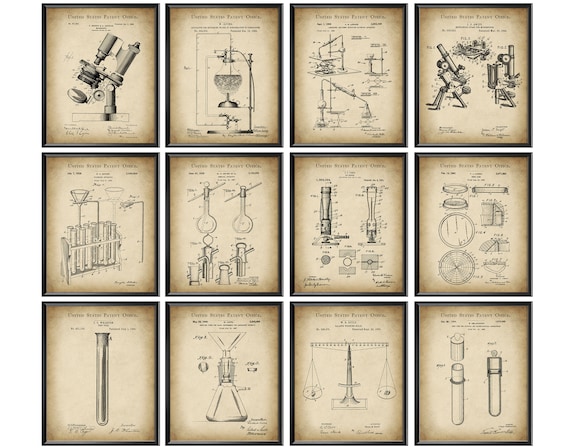The image is a compilation of 12 antique, brownish, weathered pieces of paper arranged in three rows and four columns, each with sketched or stencil-like drawings depicting various scientific inventions and apparatus. Each piece is framed by a dark brown border and separated by slight spaces. The top left image potentially illustrates a microscope, surrounded by indecipherable written descriptions. The bottom left features what seems to be a scientific beaker standing upright, while the bottom right depicts another beaker, possibly disassembled. The middle row continues with more scientific instruments, including beakers and other measurement devices, each accompanied by diagrams, numbers, and labels explaining their function. The background of each piece is darker around the edges, transitioning to a lighter center, giving the collection an antique and historical appearance.